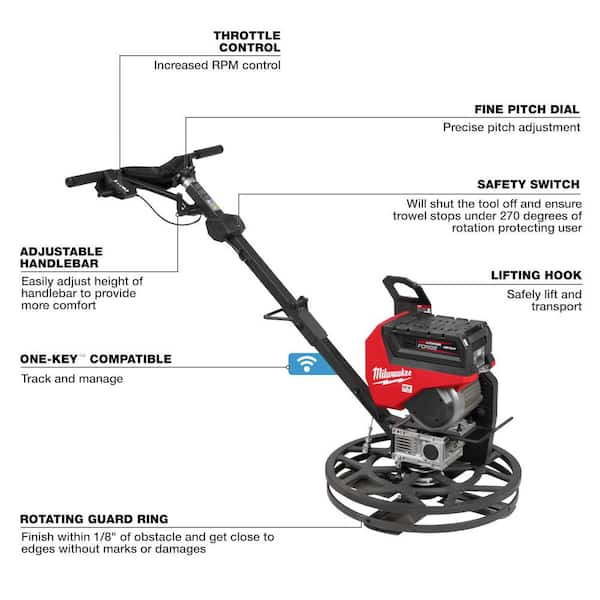The color diagram showcases a Milwaukee-branded electrical tool, likely a specialized piece of equipment such as a lawn edger or floor buffer, noted for its red and black metal body with silver accents. The tool features a long black handle with adjustable handlebars for added comfort, adorned with various operational controls. The labels detail several key components: 

- **Throttle Control**: Located on the handle to increase RPM.
- **Fine Pitch Dial**: Offers precise pitch adjustment near the handlebar area.
- **Safety Switch**: Positioned below the handle, this switch ensures the tool stops safely under 270 degrees of rotation, protecting the user.
- **Lifting Hook**: Centralized on the tool for safely lifting and transporting the device.
- **Rotating Guard Ring**: Situated at the base, it allows the tool to work close to edges without leaving marks or damages.
- **One Key Compatibility**: Highlighted for single-user operation and compatibility with multiple tools, enhancing security and manageability.

The device is set against a white background with clear labels that provide a thorough guide to its functionalities.